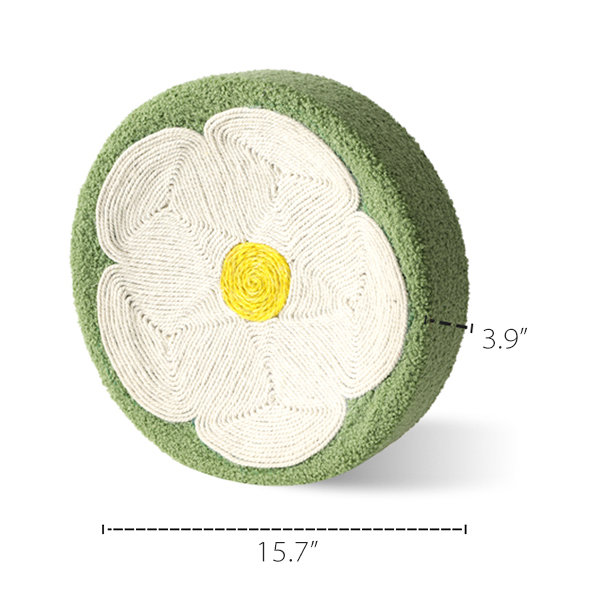The image depicts a circular, handcrafted fabric piece, measuring 15.7 inches in width and 3.9 inches in depth. The fabric appears to be a soft, nubby green material, potentially velvet, giving it a fluffy texture. At the center of this green circle is a beautifully detailed daisy design, possibly created using crochet or intricate string art. The daisy features five white petals, each meticulously detailed with intersecting stitches, and a bright yellow center, adding a visually pleasing contrast. The exact purpose of the item is ambiguous, potentially serving as a cushion cover or the top of a stool. The image also includes measurements marked with dotted lines, specifying the width and depth of the piece.